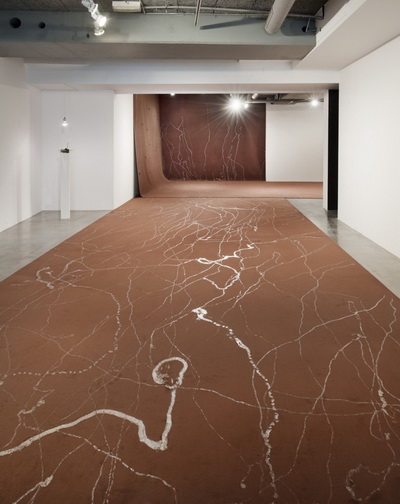This image depicts the interior of what appears to be an art gallery or museum room with wide, bright white walls bathed in foxy light. Covering three-quarters of the shiny, gray marble-like floor is a large piece of abstract art, resembling a carpet. This artwork is medium brown with streaks of what looks like white or silvery paint splattered across it, giving off an impression of an artful, random drizzle. This brown "carpet" art leads through the room toward an archway. 

Passing through the archway, the artwork continues, curving up the wall and then descending back down on the left side into a hallway. To the right of the entryway is an open black door, while a white pole with a tiny light on top stands on the left side. Beyond the arch, another section of the hallway is illuminated by a bright overhead light, casting streaks in various directions, complemented by a smaller light on the right casting a white glow. 

The room's white walls and the unique placement of the artwork contribute to an abstract, immersive experience, suggesting an environment designed to engage and provoke thought as one moves through the space.